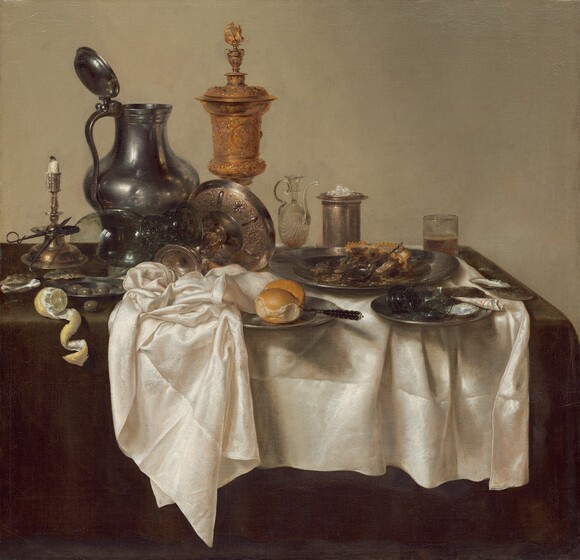This meticulously detailed painting, potentially hailing from the Renaissance period, portrays an opulent yet chaotic dinner scene on a dark wooden table. A long brown tablecloth drapes the table, partially covered by a disheveled piece of white satin cloth that bunches to the left and cascades over the right. Dominating the background is an ornate silver pitcher with its lid ajar, reflecting the dim light. In the foreground to the left, a half-melted candle sits in a brass candlestick, unlit and adding to the air of abandonment. A partially peeled lemon, its rind spiraling elegantly over the table's edge, draws the eye to the remnants of the feast. A silver plate with two dinner rolls and a knife lies prominently on the table, overshadowed slightly by a large serving platter with leftovers of a savory dish and a silver spoon. Scattered glassware, including a glass half-filled with liquid and another overturned, add to the sense of finality. The detailed illustration captures the rich textures and complex interplay of light on metal, glass, and food, set against a muted grayish-brown background. The scene evokes a narrative of opulence abruptly interrupted, leaving behind a tableau of abandoned luxury.